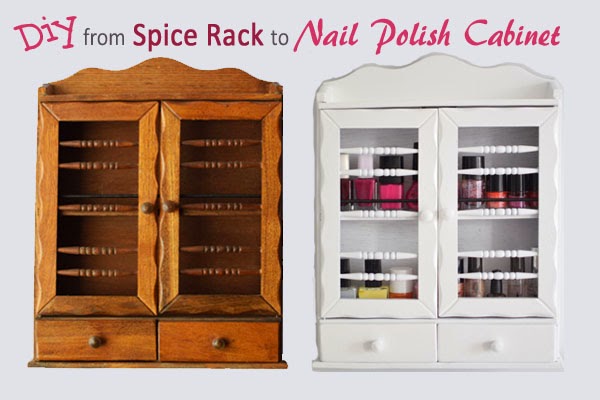The image showcases a before-and-after transformation of a vintage spice rack into a nail polish cabinet, set against a light gray background. At the top, pink text reads "DIY," followed by black text saying "from," and then dark red text that says "spicy rack," which continues in black with "to," and concludes with pink text "nail polish cabinet." On the left side, there is a small brown wooden cabinet featuring two glass-paneled doors with decorative rods, two small drawers with round knobs at the bottom, and an empty interior. On the right, the same cabinet is painted white and filled with various bottles of nail polish, neatly arranged behind the glass doors.